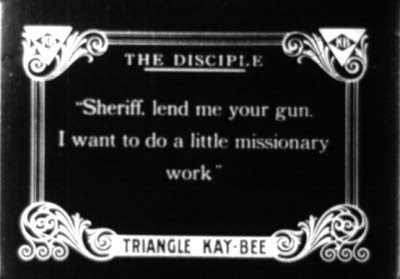The image displays a predominantly black square frame adorned with unique, white filigree designs at each corner. The top corners notably feature upside-down triangles each with a small diamond-like detail. At the top center of the frame, the title "The Disciple" is prominently written in white, underlined, and slightly fuzzy, suggesting age or slight blurriness. Directly below, the phrase "Sheriff, lend me your gun. I want to do a little missionary work." is written in the same white text. The bottom of the frame showcases a white banner with the text "TRIANGLE KAY BEE" inscribed in black capital letters. The overall ornate and slightly aged appearance of the frame contributes to its distinctive character, making the central message more poignant.